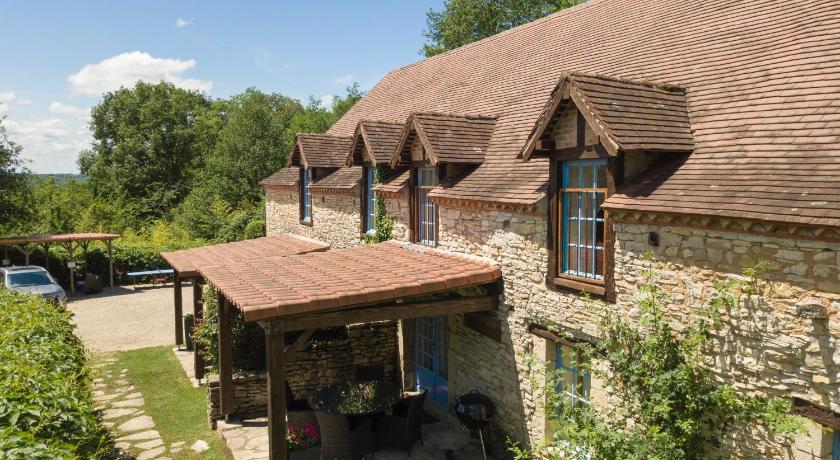This detailed photograph captures an 18th-century stone building, likely a house, characterized by its dated architecture and uneven-shaped white stonework. The two-story structure features a pitched tin-tiled roof in a brownish hue, with four dormer windows lined across the upper floor. A prominent front patio with a large roof covered in red clay tiles stands out, accompanied by a smaller adjacent tiled patio. An array of greenery adorns the scene, ranging from ivy climbing up the wall to hedges and bushes surrounding the stone path that leads to a gravel driveway, where a car is parked. Additionally, a covered parking spot can be seen. Large green trees frame the picturesque setting, under a bright blue sky dotted with big white clouds, enhancing the charming ambiance of the property.